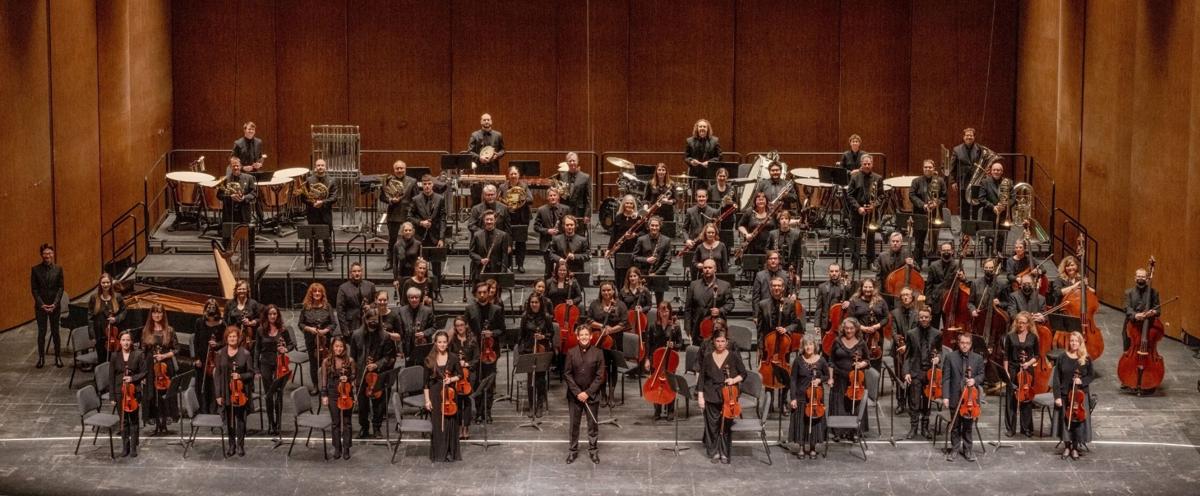This color photograph captures a full symphony orchestra assembled in a wood-paneled auditorium. Literally front and center, the smiling conductor, dressed in a black suit, holds his baton poised towards the ground. The orchestra members, also clad in black, stand in front of their chairs, holding or standing beside their instruments. The composition of the orchestra rises from the floor, with stringed instruments like violins and cellos positioned in the front rows. To the left sits the piano player, and behind them, progressively higher, are the members of the brass and percussion sections, culminating at the very top. Men and women alike, all facing forward, create an ordered yet dynamic scene, capturing the essence of their musical unity.